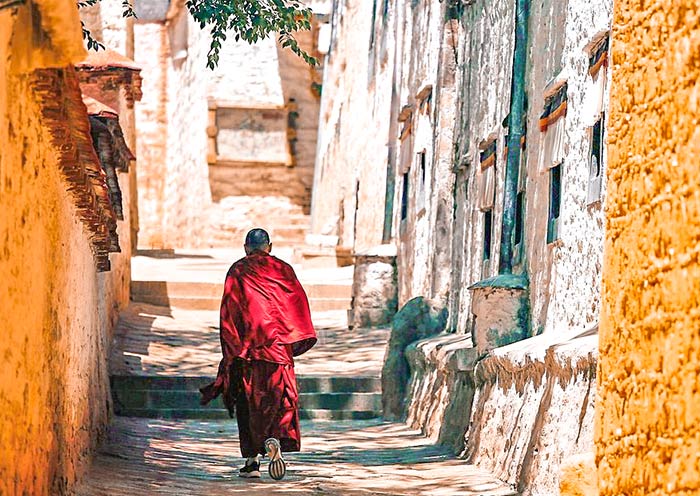In this photograph, we see a man who appears to be the Dalai Lama walking away from the camera down a narrow, ancient alley. He is dressed in traditional red monk's robes and modern sneakers, with his bald head slightly visible. The alleyway is lined with tall, cramped stone buildings on both sides, their walls a combination of weathered stone, brick, and clay with a golden-brown hue. The stone and brick structures feature white and golden-brick walls, small windows, and copper-oxidized, greenish gutters. Bright shafts of sunlight illuminate the path ahead of him, highlighting small sets of concrete steps. The first set comprises three steps, followed by a brief walkway and then an additional two steps. Vines and leaves hang from the tops of the buildings, adding a touch of green to the scene. The alleyway seems to lead toward a wall at its end, possibly indicating the entrance to a temple or another significant structure.